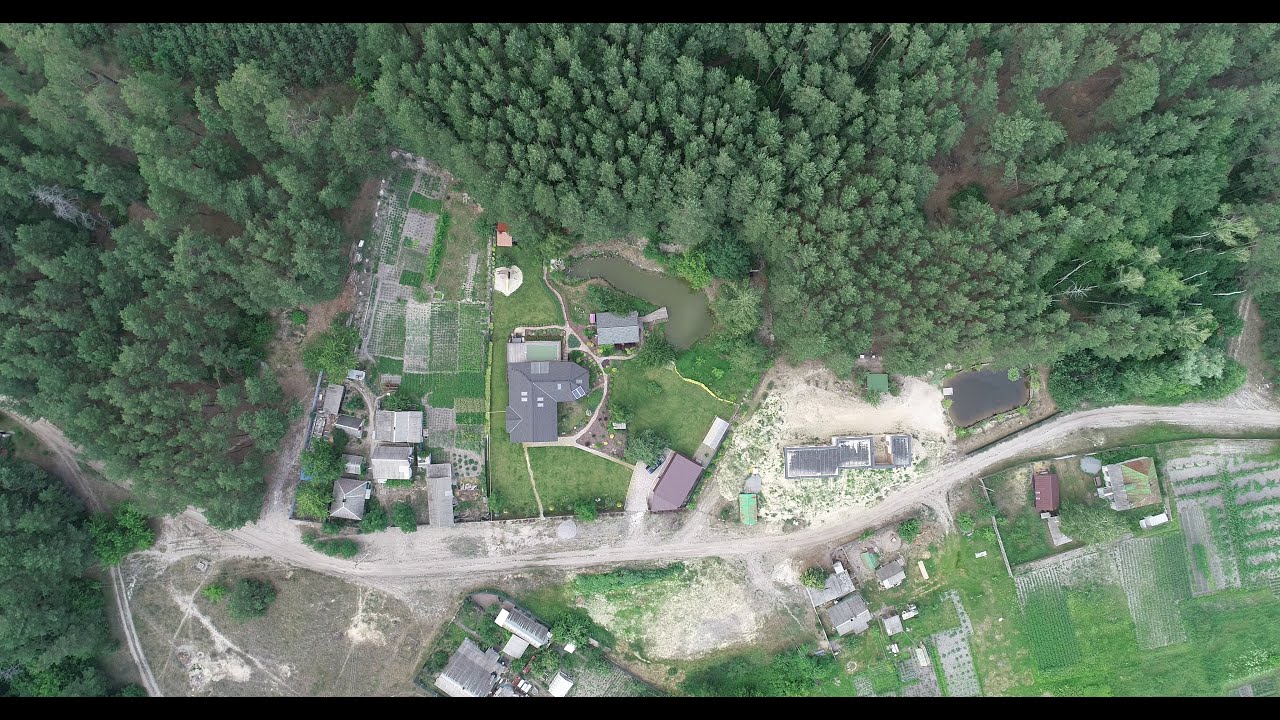This aerial image, likely captured from a high altitude via satellite or drone, showcases a predominantly green, tree-filled landscape with several clusters of buildings. The trees, which appear to include tall pine varieties, dominate the background, especially towards the upper part and left side of the image. Nestled amidst this verdant scenery are buildings with green roofs, interspersed with grassy or open areas. A light brown road runs through the scene, flanked by some of these buildings, potentially homes, and smaller structures. The road and buildings create a patchwork effect amidst the extensive tree canopy, emphasizing the harmony between the natural environment and human habitation.